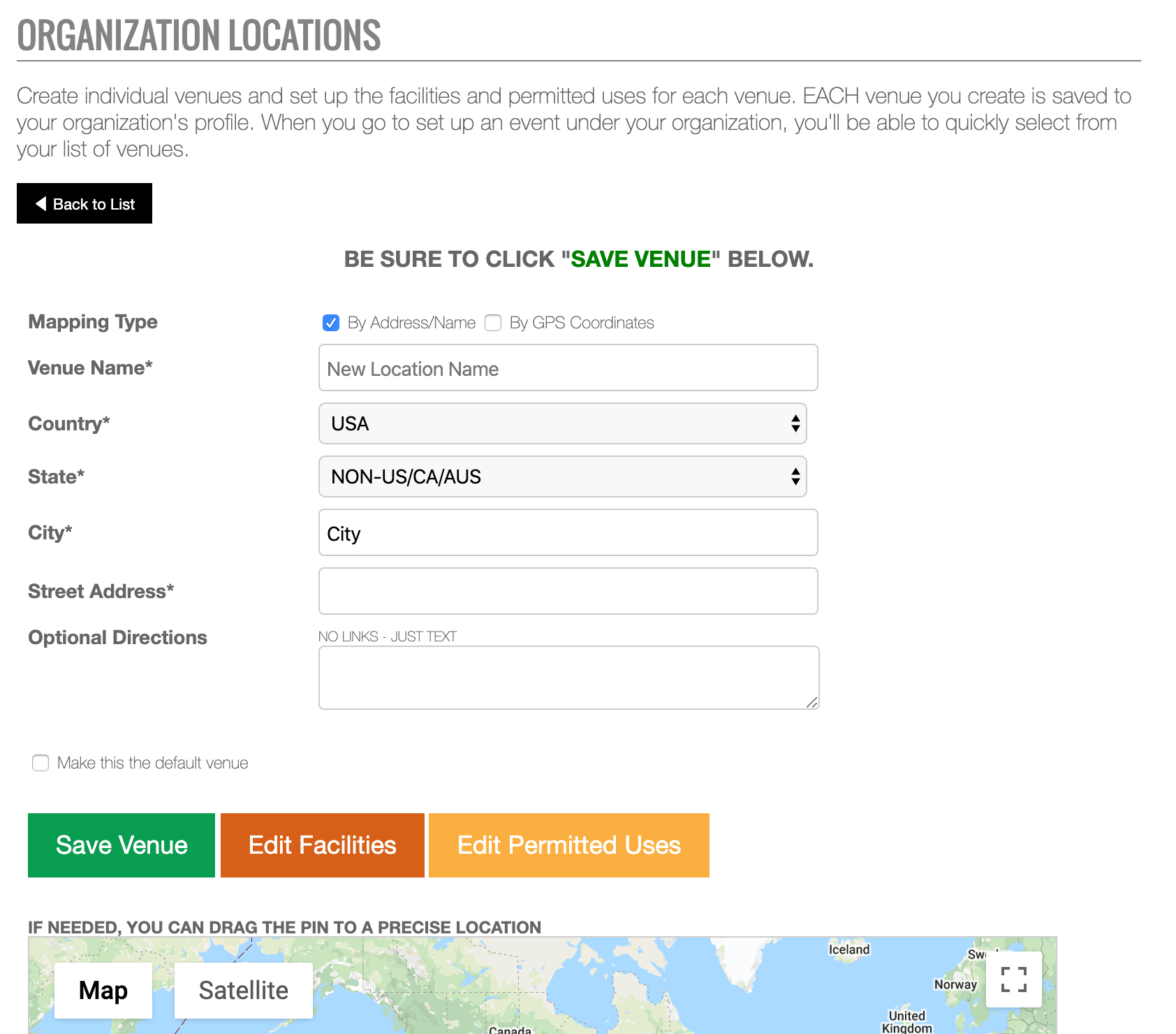The image is a square-shaped screenshot of a website interface featuring organizational information management. The title, "Organization Locations," is prominently displayed in dark gray at the top left. Below the title is a brief description followed by a small rectangular button with a black background and white text reading "Back to List." Centrally positioned within the image is an additional note in dark gray text advising users to "Be Sure to Click 'Save Venue'" with the term "Save Venue" highlighted in green.

On the left side of the image, a series of categories is listed for selecting location details. These categories include "Mapping Type," "Venue Name," "Country," "State," "City," "Street Address," and "Optional Directions." Each category is accompanied by corresponding text fields and drop-down menus for user input. The background of the image is white, creating a clean and structured layout.

Below the text fields, three buttons are visible. The first button is green with white text stating "Save Venue." The second button is red with white text labeled "Edit Facilities," and the third is orange with white text labeled "Edit Permitted Use." 

A partially visible map is located beneath these buttons. Although cut off, the map displays two gray buttons with black text providing options to view "Map" and "Satellite" modes.